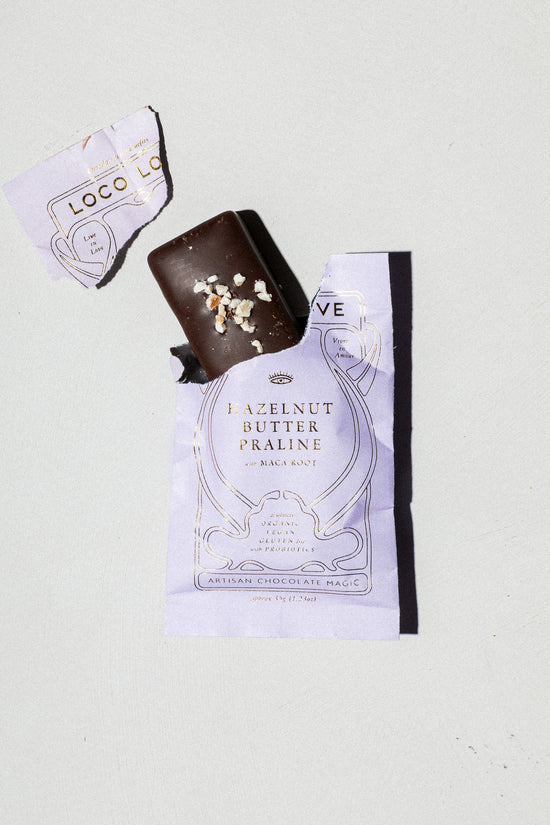The image features an opened Loco Love artisan chocolate bar on a neutral, stone-gray background. The packaging, a light lilac color adorned with silver and darker black script, has been ripped open at the top left, with the torn piece placed at an angle to the package's left. The partially exposed dark chocolate bar is sticking out at an angle, revealing a topping that includes hazelnut butter praline and possibly other ingredients like maca root. Though a shadow falls on the right side of the wrapper, the photo is well-lit, emphasizing the unique and vintage-inspired design of the packaging. The words "hazelnut butter praline" and "Loco Love" are visible, contributing to the chocolate bar’s distinct appearance.